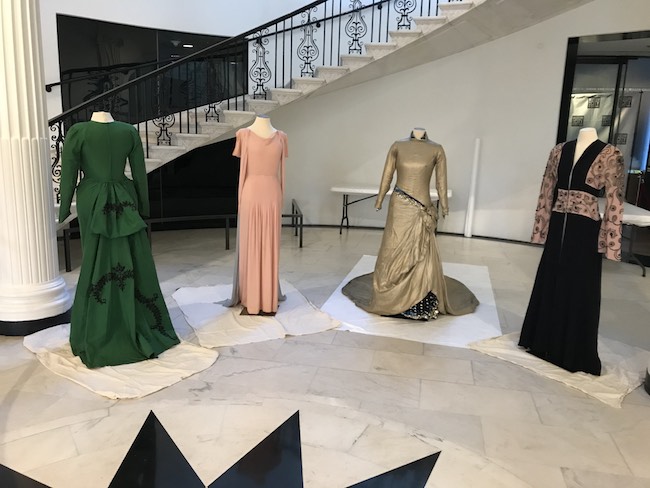In this detailed indoor photograph, a grand atrium serves as the backdrop for an elegant fashion display featuring four headless mannequins dressed in exquisite gowns. The foreground showcases an opulent marble floor, richly textured with subtle gray veining, and adorned with a rug inlaid with black triangular patterns arranged in a sunburst design. The mannequins, positioned on pristine white sheets, each showcase unique and intricate garments.

On the far left, a long-sleeve green gown impresses with a ruffled bustle, further accented with black lace detailing. Adjacent to it, a sleeveless light peach dress emanates a delicate charm with its soft flow and possibly a gentle train. The third mannequin displays a striking gold gown, featuring long sleeves, a sophisticated collar, and a dramatic ruffle pinned at the left hip, revealing black underskirt detailing. The final piece on the far right exudes an oriental-inspired elegance; the long-sleeve dress combines a black velvety skirt with bell-shaped pink sleeves adorned with intricate black patterns and a matching belt.

Behind this fashion vignette, a grand spiral staircase with ornate wrought-iron banisters arcs gracefully upwards, framed by a massive double door and a Romanesque column to the left. A wall of glass at the rear hints at another room or display area beyond the primary space, adding depth and intrigue to the scene. The overall impression is one of luxury and meticulous design, making this setting reminiscent of a high-end department store or an exclusive private residence.